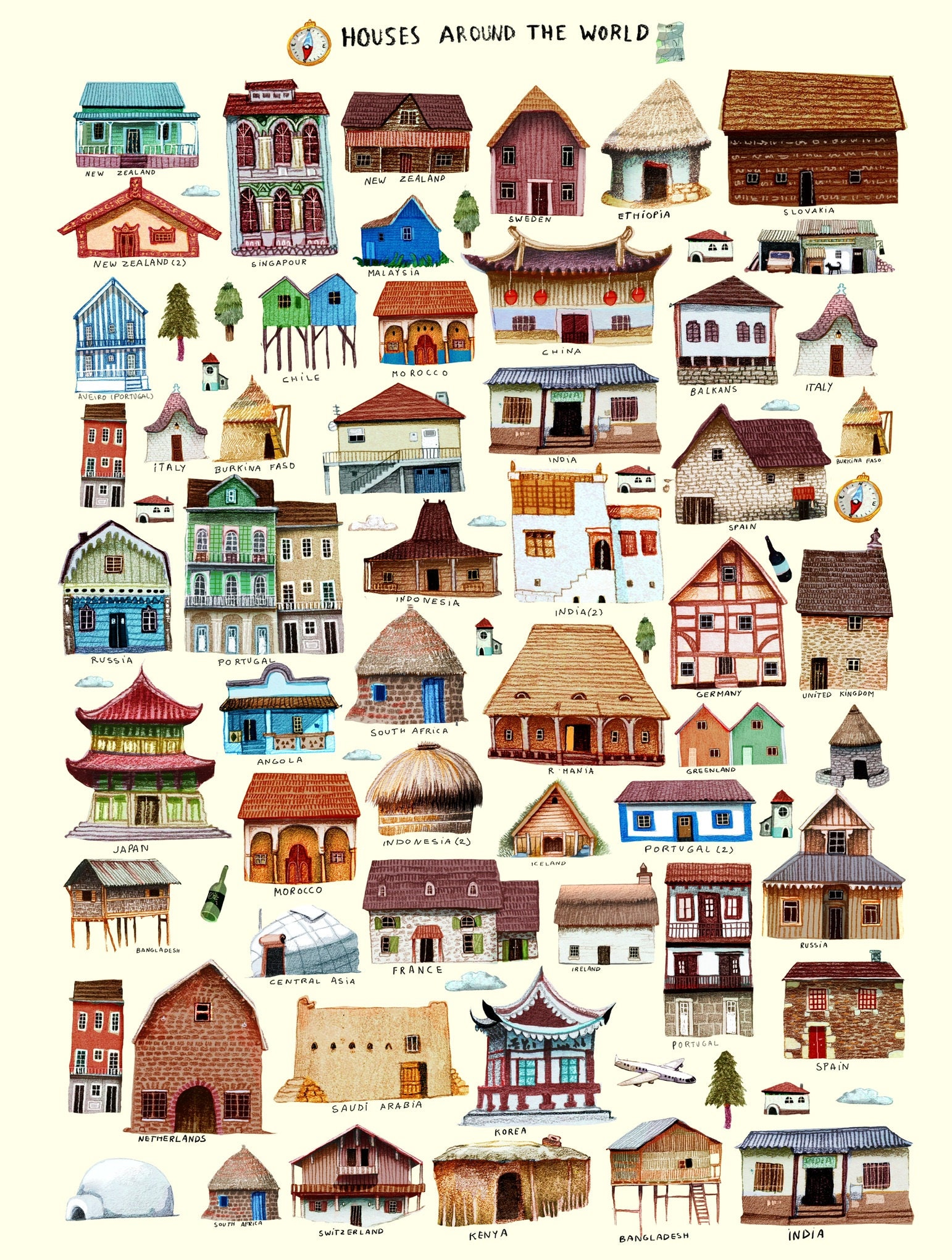The poster titled "Houses Around the World" showcases a variety of architectural styles from different countries against a tan background. The black text header at the very top reads "houses around the world." Each house is labeled with its country of origin, including New Zealand (appearing three times with one labeled as "New Zealand 2"), Singapore, Malaysia, Sweden, Ethiopia, Slovakia, China, the Balkans, Italy (appearing twice), Morocco, Chile, Portugal (appearing twice), Burkina Faso, India, Spain, the United States, the United Kingdom, Germany, and Indonesia. The poster features diverse housing structures such as sloped and flat-roofed houses, thatched-roof huts, pagoda-style buildings from Japan, barn-shaped structures typical of the U.S. Midwest, apartment buildings, log cabins built on stilts, and brick buildings. In the lower left corner, there is an igloo. Some houses have intricate designs, like Japanese pagodas with peaked tiled roofs, and others are built for practicality, such as stilt houses found in watery environments. Overall, the poster provides a comprehensive visual representation of global residential architecture.